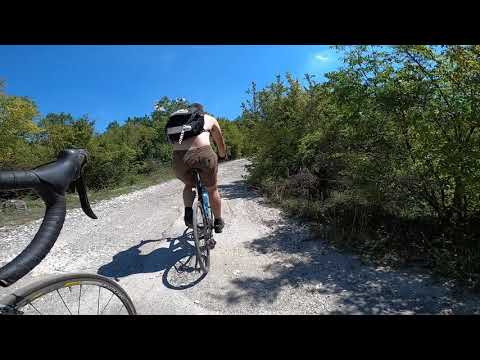In this outdoor image taken during the day, we see two cyclists navigating an uphill dirt and stone trail that curves to the right. In the lower left-hand corner, the top quarter of a bicycle tire and its black handlebars, complete with brake pads and cables, are visible, suggesting the perspective of a cyclist following behind. The main focus is on the rider directly ahead, about four feet in front; this cyclist is wearing brown shorts, socks, and shoes, and has a black backpack with a hint of white. The rider seems bare-shirted or clad in a light brown top. On either side of the trail, lush green bushes and shrubs line the path with slight scorching in some areas. The sky is a vibrant blue with minimal clouds, indicating it is likely the middle of summer. Black rectangular bars serve as horizontal borders at the top and bottom of the image.